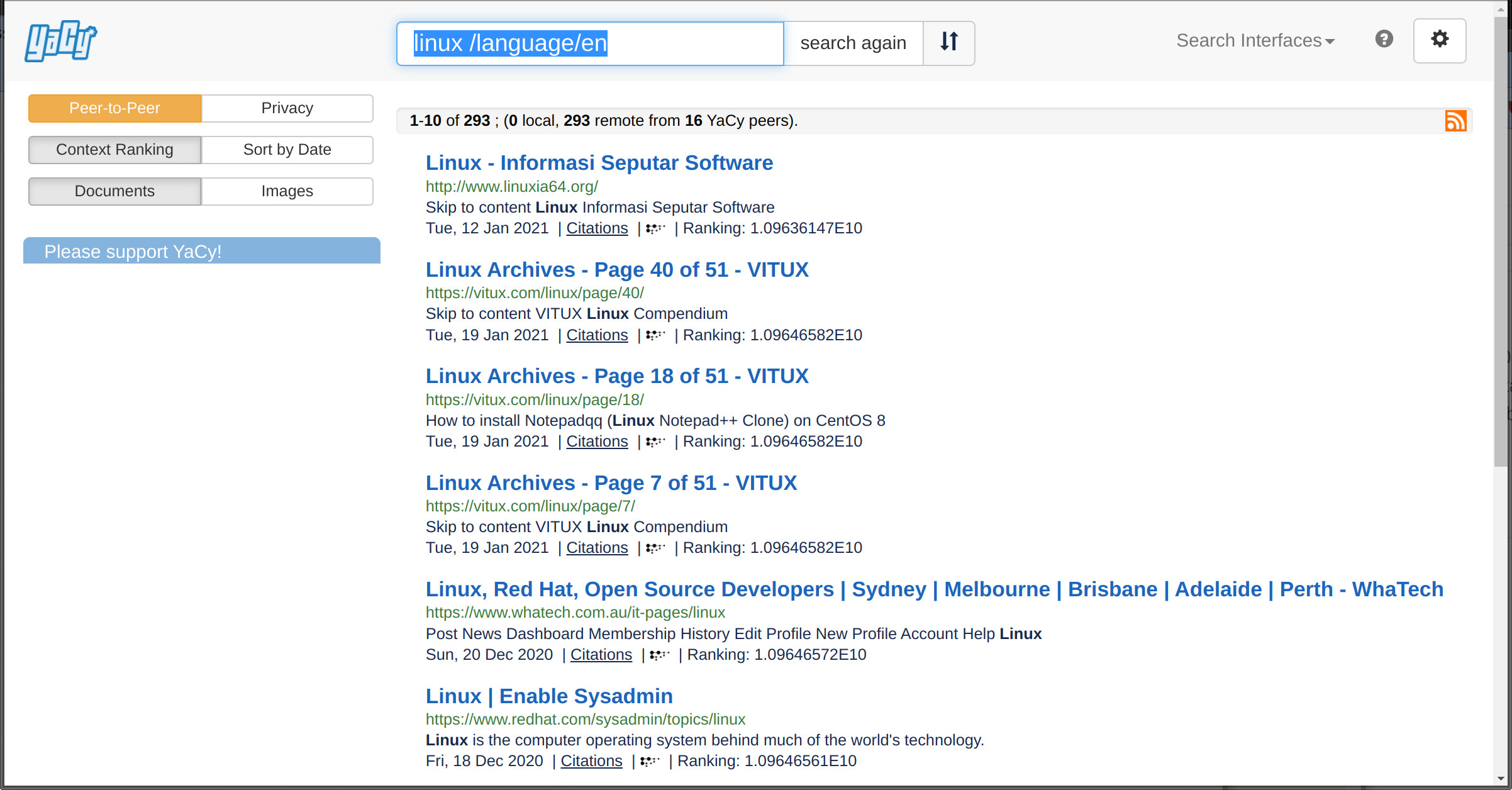The image in question is a screenshot of the YaCy search engine interface. In the upper left corner, the word "YACY" is prominently displayed in a blue-outlined font with a white fill. To the right of this, there is a search bar containing the text "Linux/language/EN," highlighted in blue with white font. Adjacent to the search bar, there is a button labeled "Search Again." On the far right side of the interface, icons for a help/question feature (a question mark inside a circle) and settings are visible.

Below the "YACY" text on the left-hand side, there is a menu containing options such as "peer-to-peer," "privacy," "contact," "rating," "sort by date," "documents," "images," and a statement encouraging users to "Please support YACY!"

In the main content area of the interface, search results are displayed, indicating that 1 to 10 out of 293 results were found, with "0 local" and "293 remote" results from 16 YaCy peers. The search results feature various information about Linux, showing excerpts like "Linux informs us simpler software," "I know no Linux IA 64.org," and links to pages such as "Linux Information and Secular Software," "Tuesday 12 January 2021 Linux Archives," and "page 40 of 51 at VITUX.com/Linux." Each result provides snippets and links, making it clear that this is a search result page for Linux-related content on the YaCy peer-to-peer search engine.